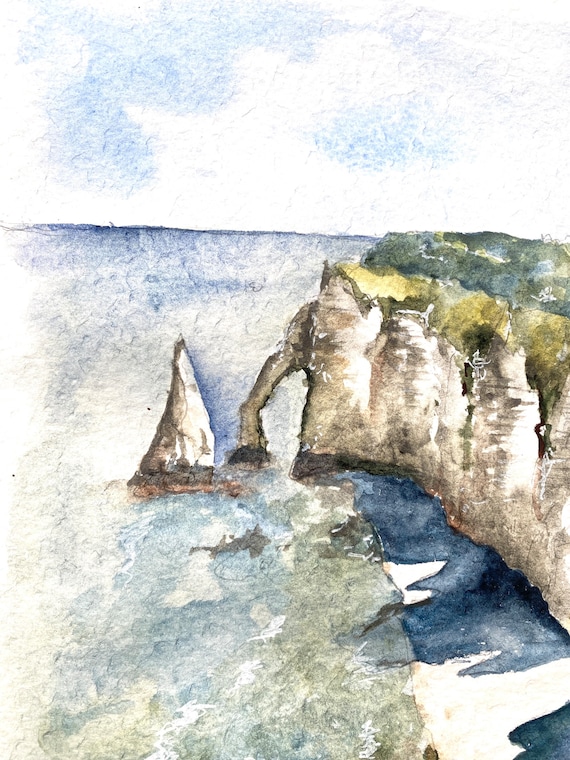This image depicts an abstract watercolor painting of a seascape with a prominent rocky cliff. The sky at the top of the painting features subtle shades of light blue intermingled with white. The ocean below stretches across the canvas, transitioning from dark blue in the distance to varying hues of green and light blue towards the foreground. On the right side of the image, a jagged rock formation, shaded in brown and accented with white, rises next to the water. Atop the cliff, there's a hint of greenery comprising trees and grass. Near the base of the cliff, there is an indistinct, triangular shape in the water, which seems to be a small sailboat with a tall white sail. The water's rough texture is evident from the brushstrokes, adding to the dynamic feel of the scene. Despite its abstract and less detailed style, the painting evokes the essence of a coastal landscape.